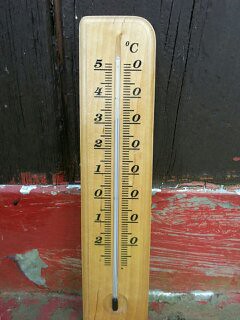In this photograph, a wooden backdrop is prominently featured, comprised of two distinct sections: a black-painted upper portion and a red-painted lower portion. The black section, which occupies approximately two-thirds of the backdrop, appears freshly painted but visibly worn, revealing natural divots and cracks beneath the paint. In contrast, the red section, occupying the bottom third and connecting to the floor, shows signs of age with peeling and chipped paint.

Leaning against this dual-colored wooden backdrop is a thermometer calibrated in Celsius. The thermometer is marked with temperature readings ranging from -2 to 5 degrees Celsius. On the right side, all readings are set to zero, while the left side displays incremental values: 5 at the top, descending to 4, 3, 2, 1, 0, and then continuing to -1 and -2. The current temperature is indicated at 3 degrees Celsius on the left side and 0 degrees Celsius on the right side.